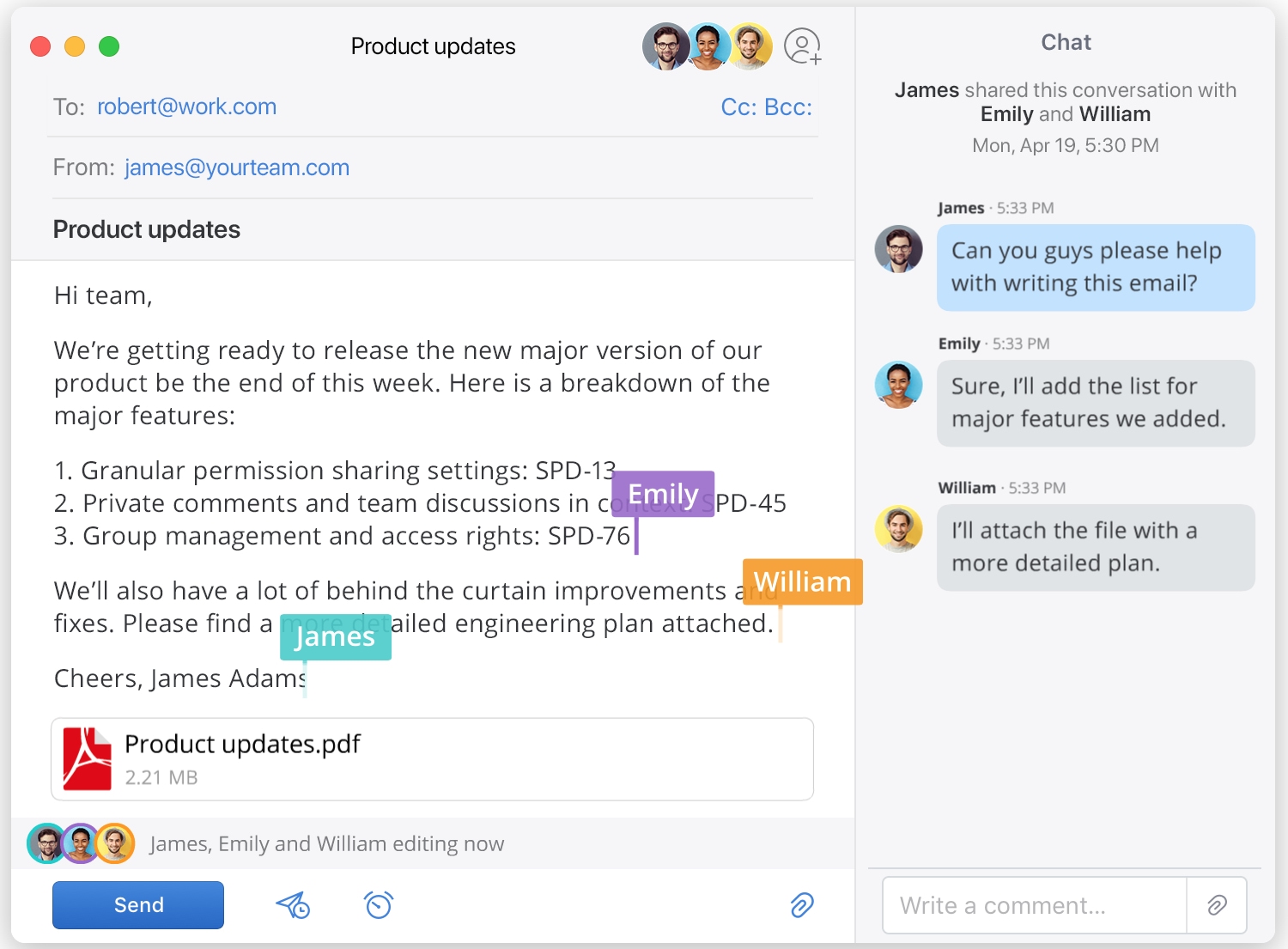The image depicts an active screen where an individual is composing an email about product updates. The scene is divided into two sections: on the left, the draft email is visible, and on the right, a chat window shows an ongoing conversation among colleagues, namely James, Emily, and William.

In the chat window, James initiates the discussion by asking, "Can you guys please help with writing this email?" Emily promptly responds, "Sure, I'll add the list for major features we added," followed by William stating, "I'll attach the file with more detailed plans."

The email being drafted reads as follows:
"Hi team,
We're getting ready to release the new major version of our product by the end of this week. Here is a breakdown of the major features:
1. Granular permission sharing settings
2. Private comments and team discussions
3. Group management and access rights
We'll also have a lot of behind-the-curtain improvements and fixes.
Please find the detailed engineering plan attached.
Cheers,
James Adams"

In the email draft, contributions from James, Emily, and William are clearly visible. Additionally, there is a PDF attachment titled "Product Updates" appended at the end of the email. 

This detailed depiction emphasizes the collaborative effort involved in crafting the email and highlights the specific roles each colleague played in its formulation.